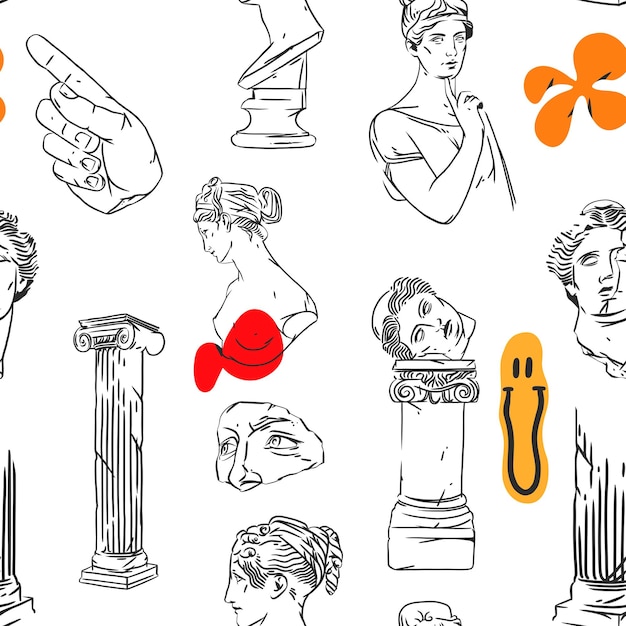The image depicts a detailed black-and-white ink drawing on a solid white background, roughly square in shape. Scattered throughout the picture are various sketches, leaning heavily on themes of Roman architecture and classical art. Among the illustrations, there are five prominent head busts and three distinct columns. Additionally, there are sketches of a hand with its index finger pointed, a foot resting on a pillar, and a peculiar representation of a person with their pointer finger under their chin. There's also a disembodied head placed on top of a column, just the eyes and nose of a face, and a side profile of a woman with her hair styled in an updo. Some parts of the statues depicted appear cracked or incomplete. The drawing features vibrant spots of color: a noticeable yellow blob with a smiley face towards the center-right, a red mark on one of the busts, and an orange blotch resembling a flower petal at the top right. The surreal combination of classical sketches and random blobs of color gives the image a strange yet amusing appearance.